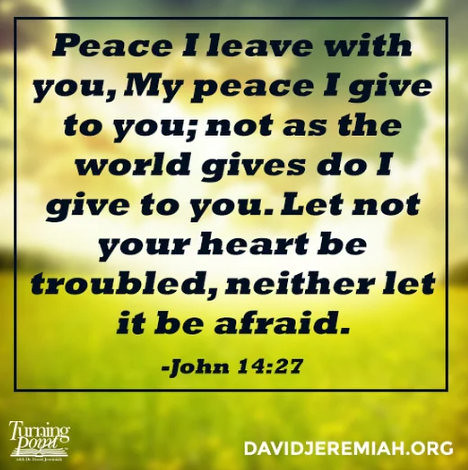The image features a motivational religious message drawn from the Bible, specifically John 14:27, likely from the King James version. The quote, "Peace I leave with you, my peace I give to you; not as the world gives do I give to you. Let not your heart be troubled, neither let it be afraid," dominates the majority of the image. In the bottom left corner, the logo "Turning Point" is displayed in white text, while on the bottom right, the URL "DavidJeremiah.org" appears in capital white letters. The background consists of a slightly blurred green field with distant trees on both sides, under a sky filled with gray and white clouds against a blue backdrop. The image employs a soft color palette featuring greens, whites, blacks, and grays, creating a peaceful and reflective atmosphere designed for online sharing.